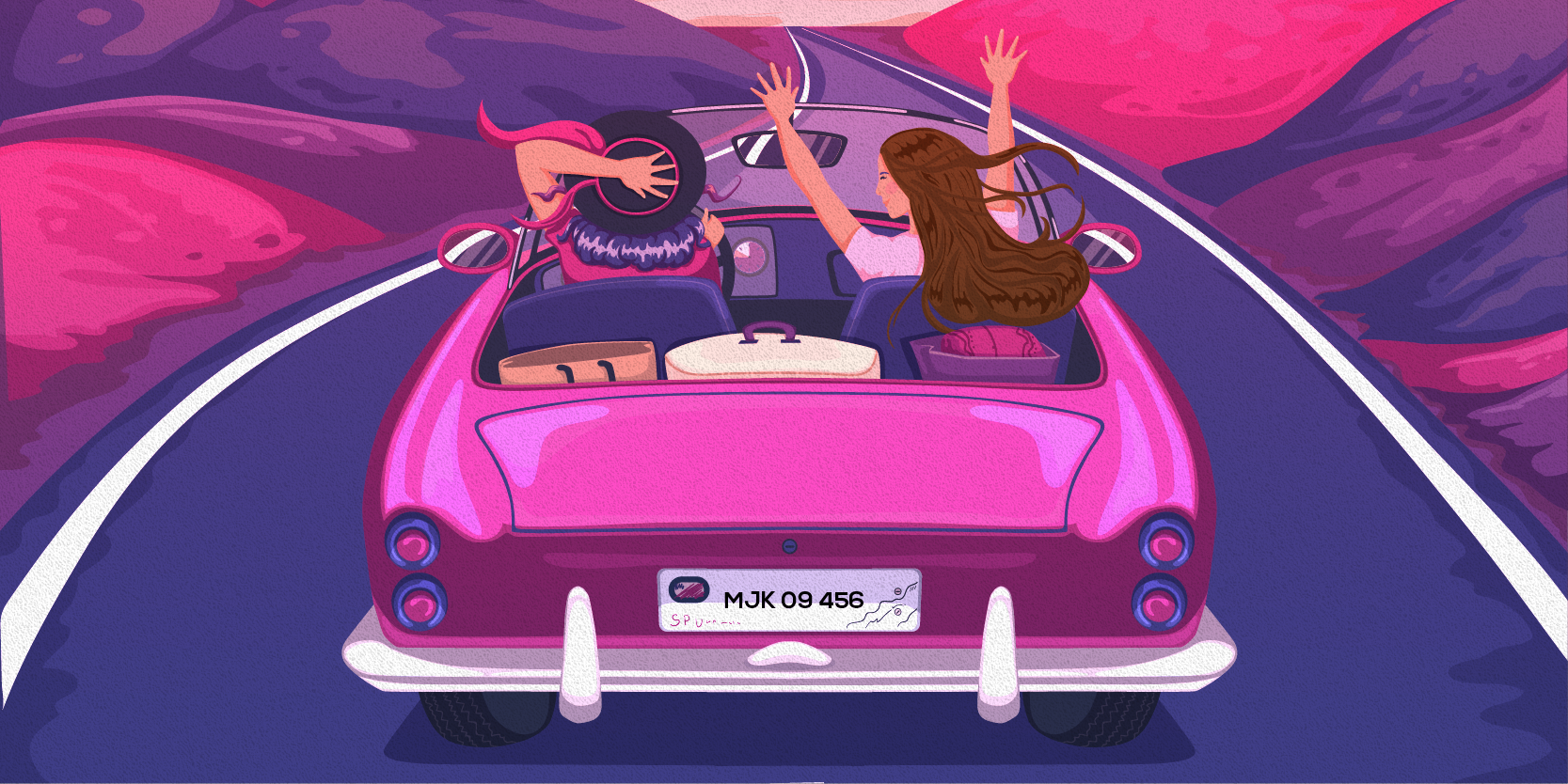The image depicts a cartoon-like, anime-inspired drawing of two women driving a pinkish-purple convertible with the roof down on a visually striking purple asphalt road. The car is moving away from the viewer, down the center of the image, flanked by solid white road lines. The landscape on both sides of the road features vibrant, slope-like formations in shades of pink, purple, and dark purple, devoid of any greenery.

The vehicle itself is meticulously detailed with four rear purple taillights, white rear bumper, black tires, and a prominent rectangular white license plate bearing the number MJK09456 in black letters. The car’s interior is predominantly purple, including the seats, dashboard, and windshield. The rearview mirrors are pink and purple.

In the backseat of the convertible are multiple bags, suggesting a shopping trip. One is a brown purse with a black strap, another resembles a white hamper with a purple handle, and the last one is a purple bag containing a pink item.

The two women in the car exude a carefree vibe. The driver has purple hair, wears a black hat with a pink ribbon, a pink shirt, and grips the steering wheel with one hand while holding her hat with the other. The passenger, with long brown hair, appears animated with her hands in the air and is dressed in a white shirt. The surreal, high-contrast hues of pink and purple dominate the entire scene, making it an eye-catching and whimsical visual journey.